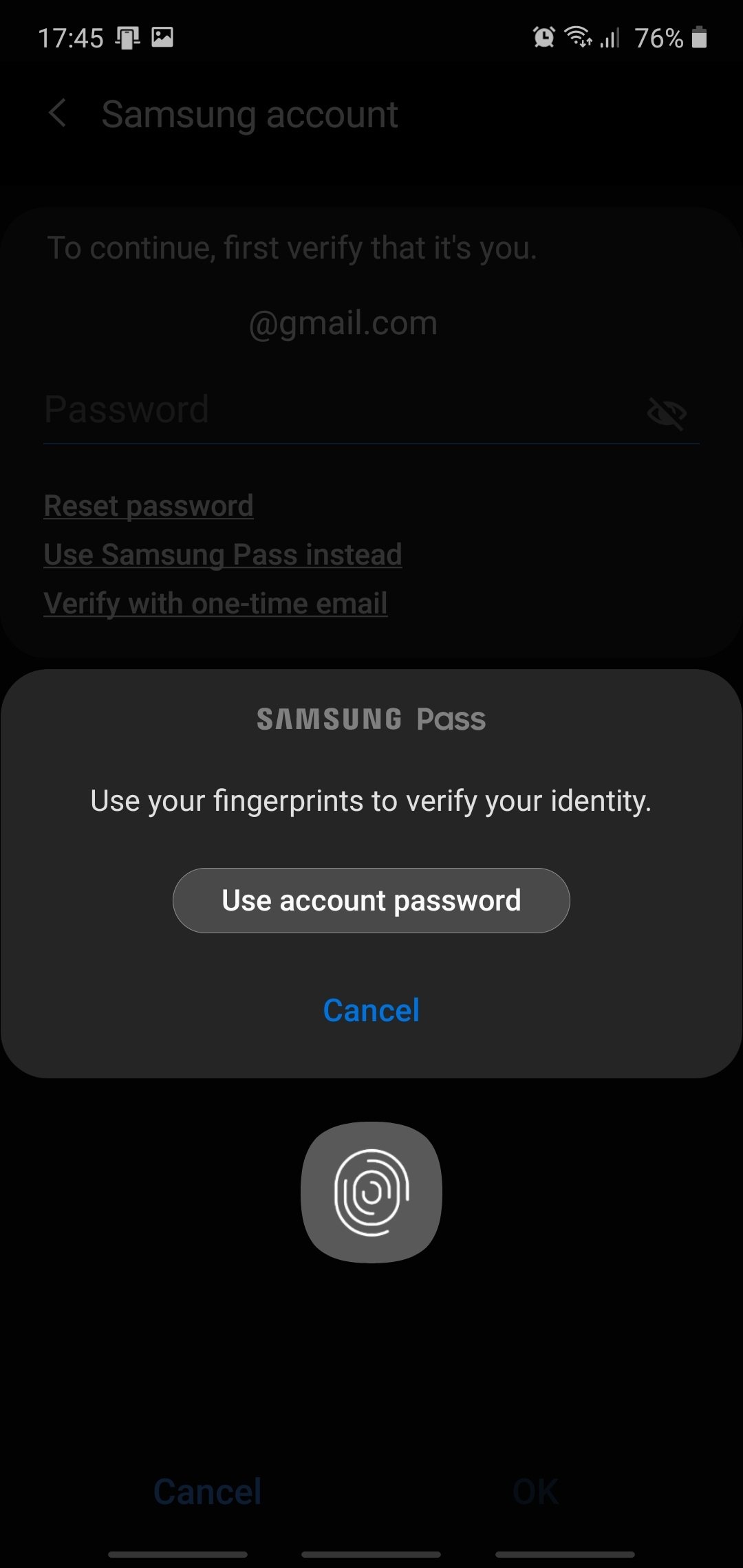**Detailed Caption:**

The image portrays a black rectangular screen with various interface elements layered across it. At the top center, the time "17:45" is displayed in white text. Below this, the screen content appears to illustrate a login or verification interface, potentially for a Samsung device.

On the right side of the interface, there are several icons and indicators:
- An alarm clock symbol.
- A Wi-Fi signal strength indicator composed of four lines that increase in size from left to right. Three of these lines are white, while the fourth is gray.
- A battery icon indicating a 76% charge level.

In the main body of the screen, gray text reads, "Samsung account," and an arrow pointing left is visible. Below this, the interface prompts the user with "To continue, first verify that it's you," followed by an email address ending in "@gmail.com". The email text suggests there’s an input field provided for the user to enter their credentials.

Further down in the interface, extremely dark gray text indicates an entry for a password, accompanied by a symbol resembling an eye with a slash through it, suggesting an option to show or hide the password. Underneath the password field, a dark gray line extends horizontally.

Additional options presented in lighter gray text include "Reset password," "Use Samsung Pass instead," and "Verify with one time email."

A light gray rectangular button with rounded corners reads "Samsung Pass: Use your fingerprint to verify your identity." Directly below this, another lighter gray rectangle is slightly bulged at the sides and states "Use account password."

Near the bottom of the screen, to the left, the word "Cancel" appears in blue text. To the right, a greyed-out square with rounded corners contains a fingerprint icon. Finally, at the very bottom in faint text, "Cancel" appears in blue on the left, while "Okay" is hinted at on the right, and three horizontal gray lines are visible, possibly representing further options or settings.